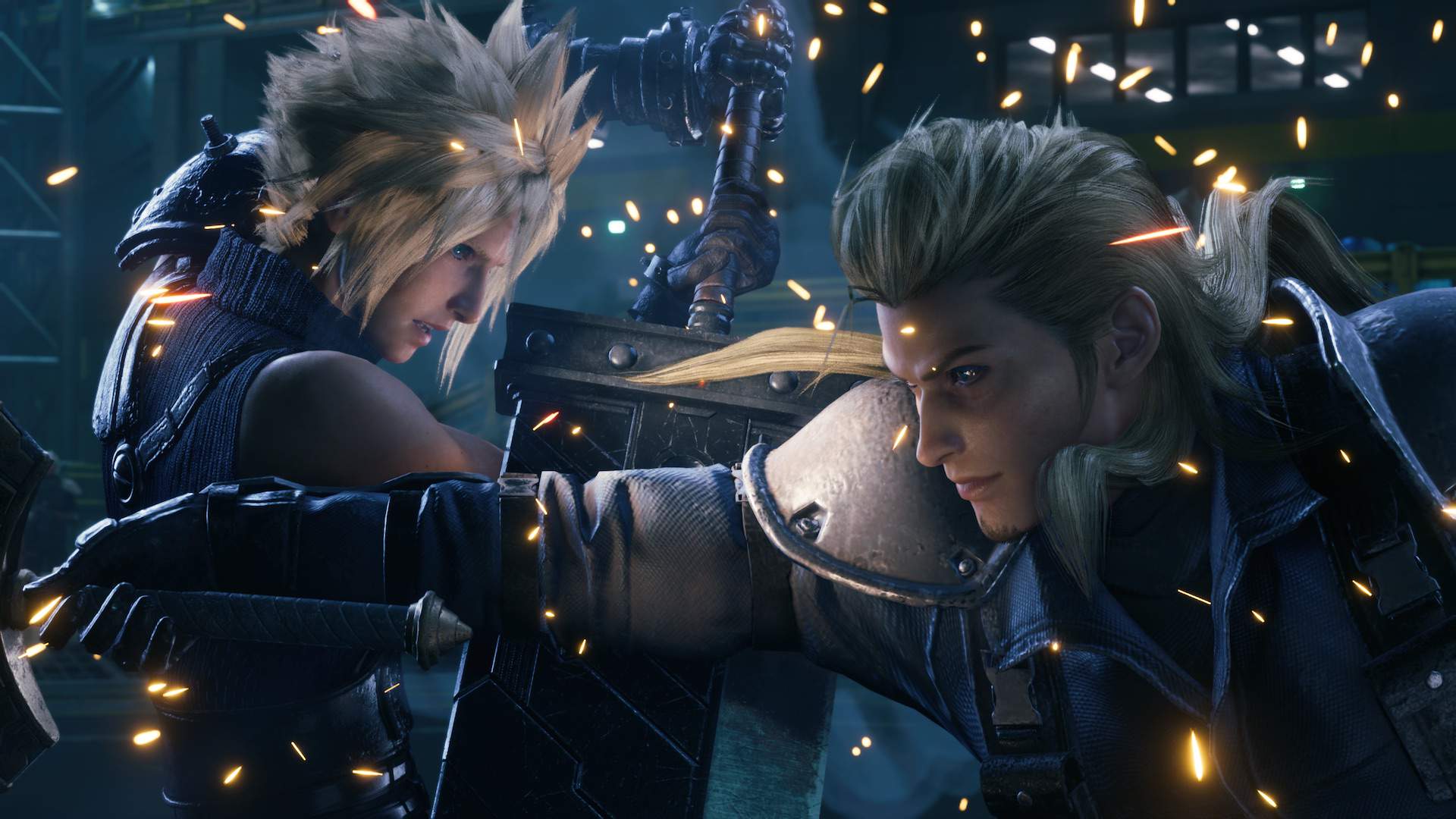The image is a dark, computer-rendered 3D scene of a combat between two warriors, set in what appears to be nighttime. The female figure on the left has striking, spiky blonde hair and wears a sleeveless turtleneck sweater with black gloves, wielding a sword. The male figure on the right, also with blonde hair, is clad in a combination of a blue pullover and intricate gray and silver armor. Both fighters are surrounded by fiery sparks flying through the air amidst a dark, obscured background, suggesting intense action. The woman is positioned slightly behind and to the left, looking back to the right, while the man stands in the foreground, facing slightly left. The scattered blips of light around them add to the high-energy and chaotic atmosphere of their confrontation.